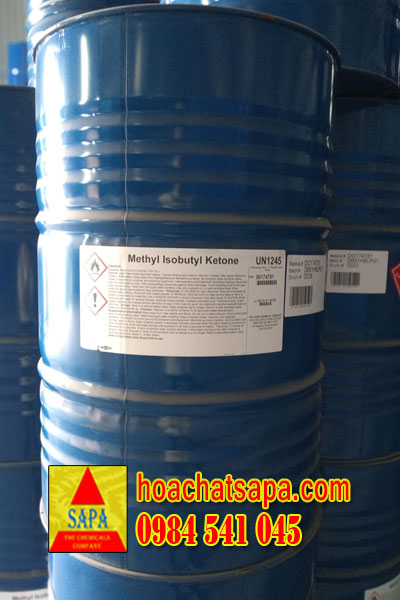The image features a tall, metallic blue canister prominently in the center, with similar canisters in the background. The canister bears a label with a variety of information. At the top of the white label, in large bold black text, is the chemical name "Methyl Isobutyl Ketone," accompanied by "UN 1245" on the top right. Just below this text, to the left, are two diamond-shaped hazard symbols: one indicating flammability and the other showing an exclamation mark, signaling caution. Centrally positioned on the label is a bar code with another bar code sticker to the right. At the bottom of the label, the logo of the chemical company, SAPPA, appears within a red triangle on a yellow background. Beneath the logo is the company’s contact information, written in blue text as "hoachat@sappa.com" along with the phone number, "0984541045." The image's background is indeterminate, with the main focus being entirely on the detailed depiction of the chemical canisters. The lighting comes from the left side, casting a highlight across the canister, and suggesting a setting such as a product advertisement or an industrial catalog.